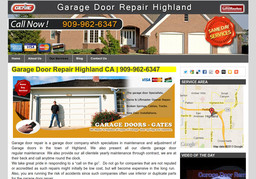A small, square-cropped image advertising a garage door repair company. At the top, a gray header features bold white capital letters that read "Garage Door Repair Highland." To the left of the text is an out-of-focus red circle with white font, likely the company logo. On the right side, a rectangular red box with white text is also out of focus. Below the header, a large photo shows the front of a house, focusing on the garage door. The top left of this photo has a gray banner with "Call Now" in large white letters and a phone number in large yellow digits.

At the bottom left of the photo, icons for American Express, Visa, and MasterCard are displayed. To the far right, a wax stamp clipart with the phrase "Same Day Services" is visible in yellow font. 

A highlighted section at the bottom of the image reads "Garage Door Repair Highland California," with the phone number below. To the left, another large box with a photo background shows a man standing in front of a garage door. On the right side of this box, a square section contains a map graphic.